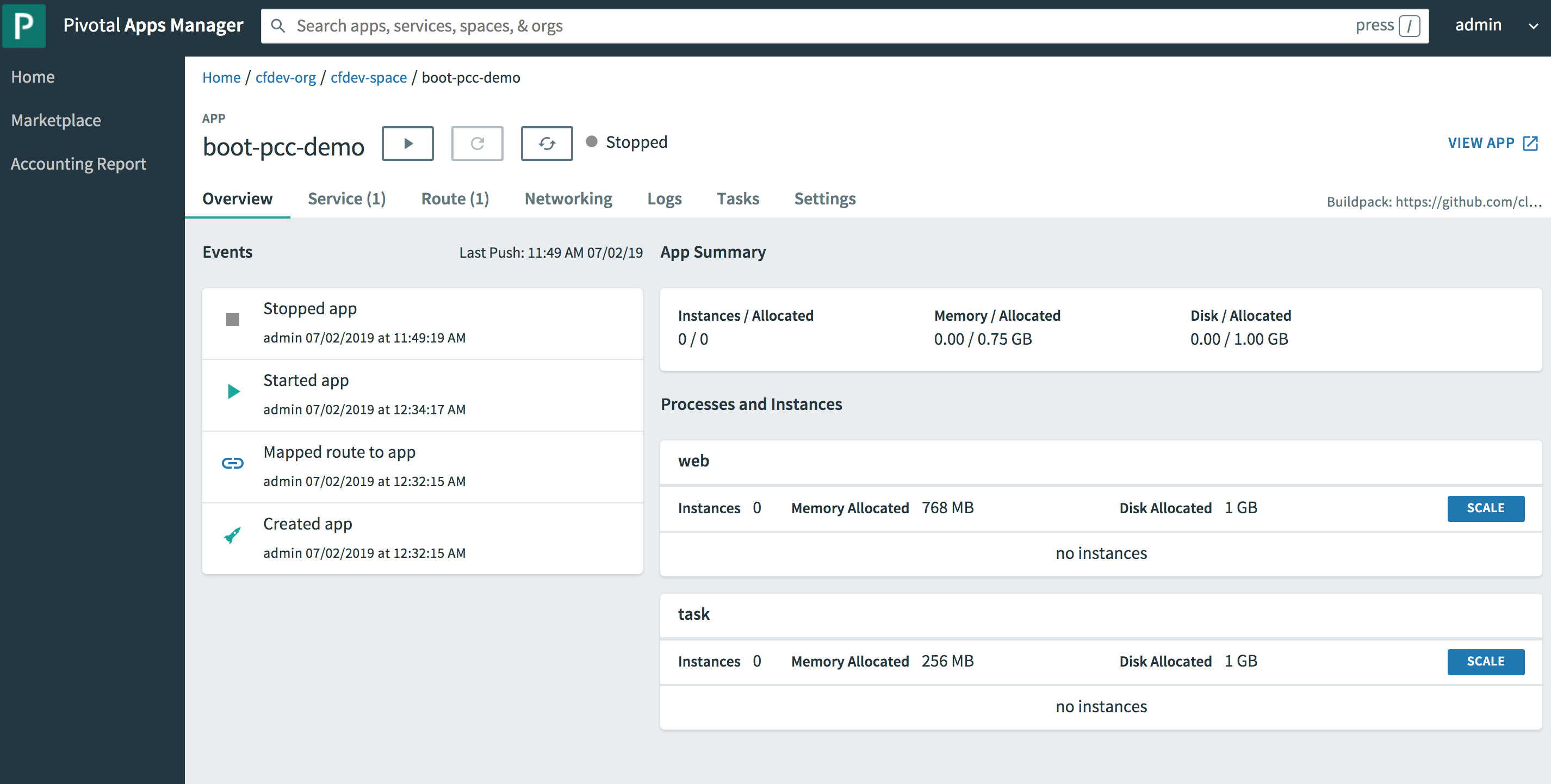The image depicts the Pivotal Apps Manager interface. Dominating the top left corner is a prominent letter "P," accompanied by a green box with a white "P" inside, signifying the Pivotal logo. To the right, a search bar labeled "search apps, services, spaces, and orgs" hints at its functionality for navigating through different entities. A user prompt indicating that pressing the forward slash key may modify search behavior is also present.

The user appears to be logged in as an administrator, as evidenced by the "admin" label in the drop-down menu located at the top right of the interface. On the left, a sidebar displays various navigation options, including "Home," "Marketplace," "Accounting," and "Report."

The main page features a breadcrumb path showing the current location within the system hierarchy: "Home / CD CF Dev / Boot PCC Demo." The central content area is populated with various technical details about the application environment, including information about instances, tasks, root mappings, and disk allocation space.

Overall, the interface seems designed to facilitate the management of multiple applications, potentially including different versions such as beta or alpha releases. The detailed technical information displayed likely aids in the administration and monitoring of these applications.